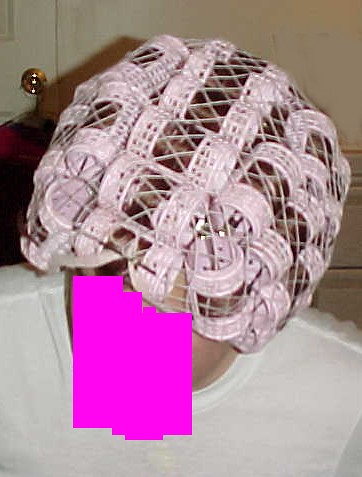The photograph is an indoor, horizontally-oriented, color image with a grainy, slightly out-of-focus quality suggesting it may have been taken in the 1980s. The scene features a close-up view looking down on what appears to be a woman's head, which is covered with about 15 to 16 pink hair curlers arranged symmetrically. Her brunette hair is secured under a white hairnet. The face in the image is obscured by crude purple or pink digital strokes or tape, forming a semi-square shape. She is wearing a white, almost featureless t-shirt. In the background, there is a white cabinet with brass knobs, one of which has something hanging on it. The overall setting includes a white counter or sink area. No text is present in the image, and the lighting is bright yet contributes to the slightly low-resolution quality of the photograph.